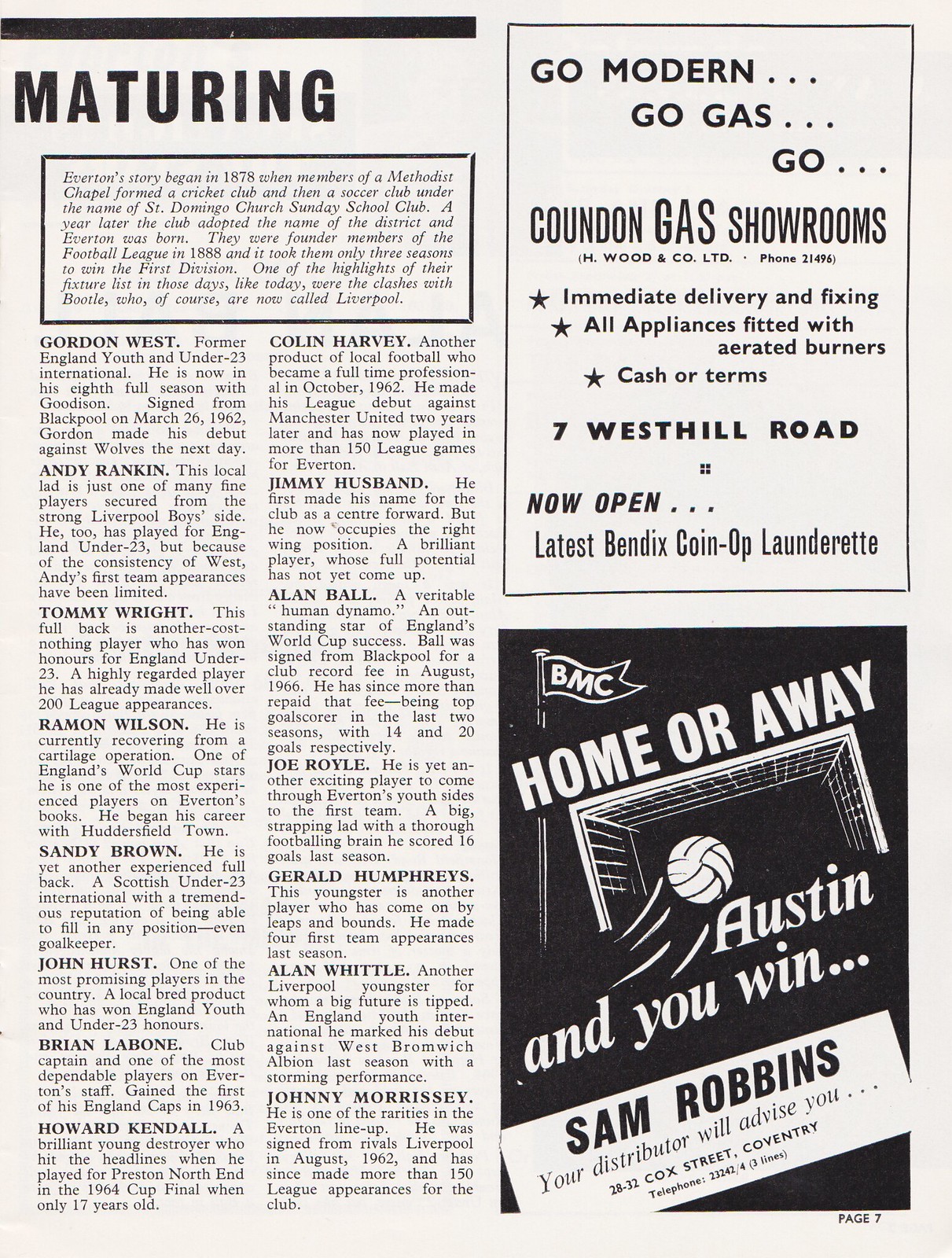The image depicts a newspaper or magazine advertisement article. On the left side, in bold black text, is a column titled "Maturing," which features detailed descriptions of various sports team members, listing names like Gordon West, Andy Rankin, Tommy Wright, Ramon Wilson, Sandy Brown, John Hurst, Brian Lebone, Howard Kendall, Colin Harvey, Jimmy Husband, Alan Ball, Joe Royal, Gerald Humphreys, Alan Whittle, and John Morrissey. This section includes biographical snippets about the players, such as Colin Harvey, who became a full-time professional in October 1962 and made his league debut against Manchester United, amassing over 150 league games for Everton.

On the right side of the image, there are two black and white advertisements bordered prominently and occupying a significant portion of the page. One ad promotes a showroom, while the other features a slogan at the bottom right, "Home or Away Austin and You Win," accompanied by an illustration of a soccer ball scoring a goal. Both sections are visually separated with borders around the text and ads, ensuring the content is clearly defined and organized.